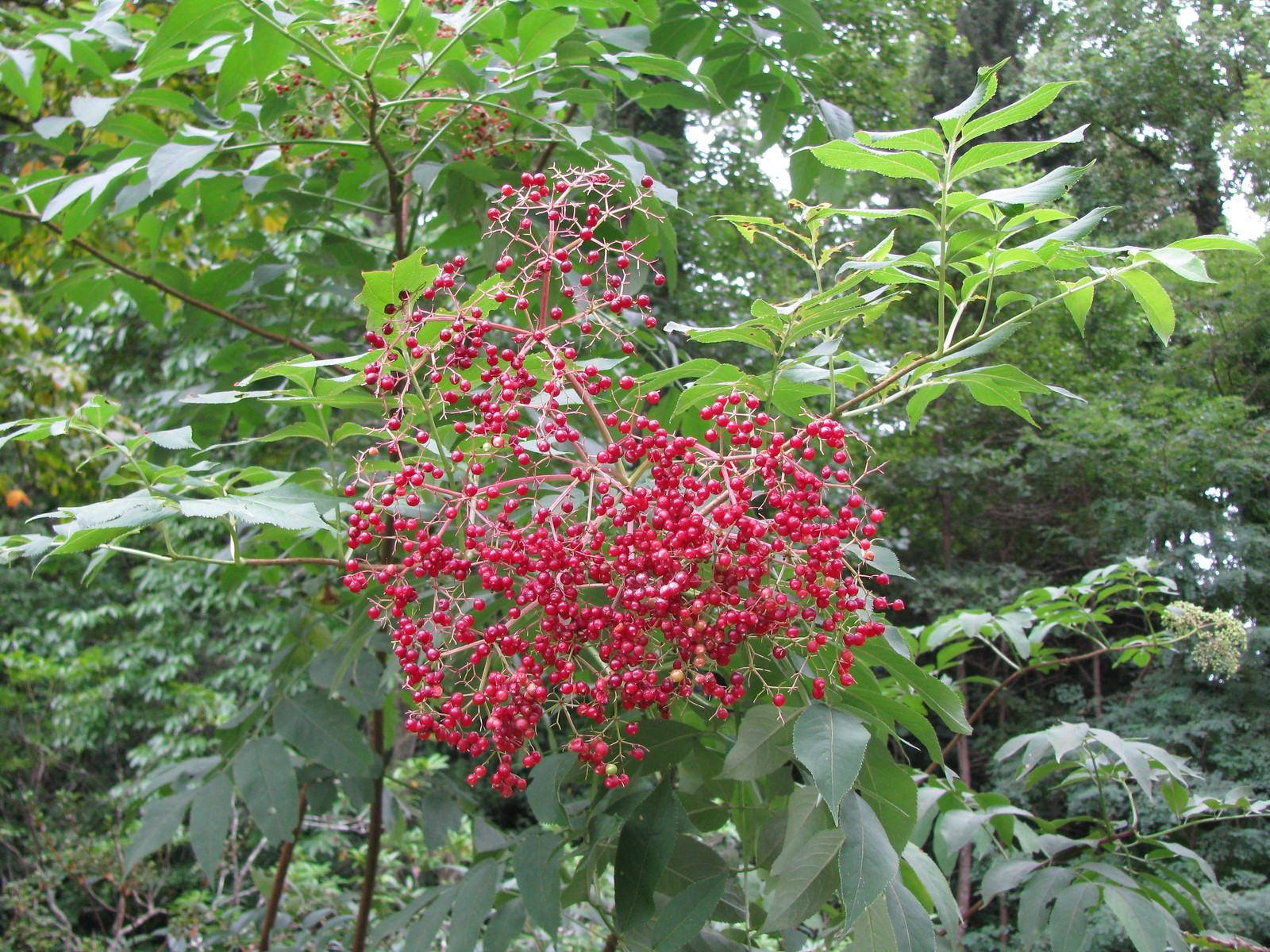This wide rectangular image captures a detailed outdoor scene centered on a bush filled with clusters of tiny red berries, most densely packed at the bottom of the branches. These branches emerge green but gradually turn red and spread out in numerous directions, adding a visual depth to the arrangement. The bush is set against a backdrop of green stems with floppy, triangular leaves, creating a lush green environment. Farther in the distance to the right, towering trees with slightly darker green leaves rise up, contributing to the layered greenery of the scene. At the bottom of the photo, there is a cluster of shadier, more grayish-green leaves. The atmosphere suggests a somewhat cloudy day, hinting at an overcast sky, which casts a soft, diffused light over the scene, enhancing the natural vibrancy of the red berries and rich greenery surrounding them.